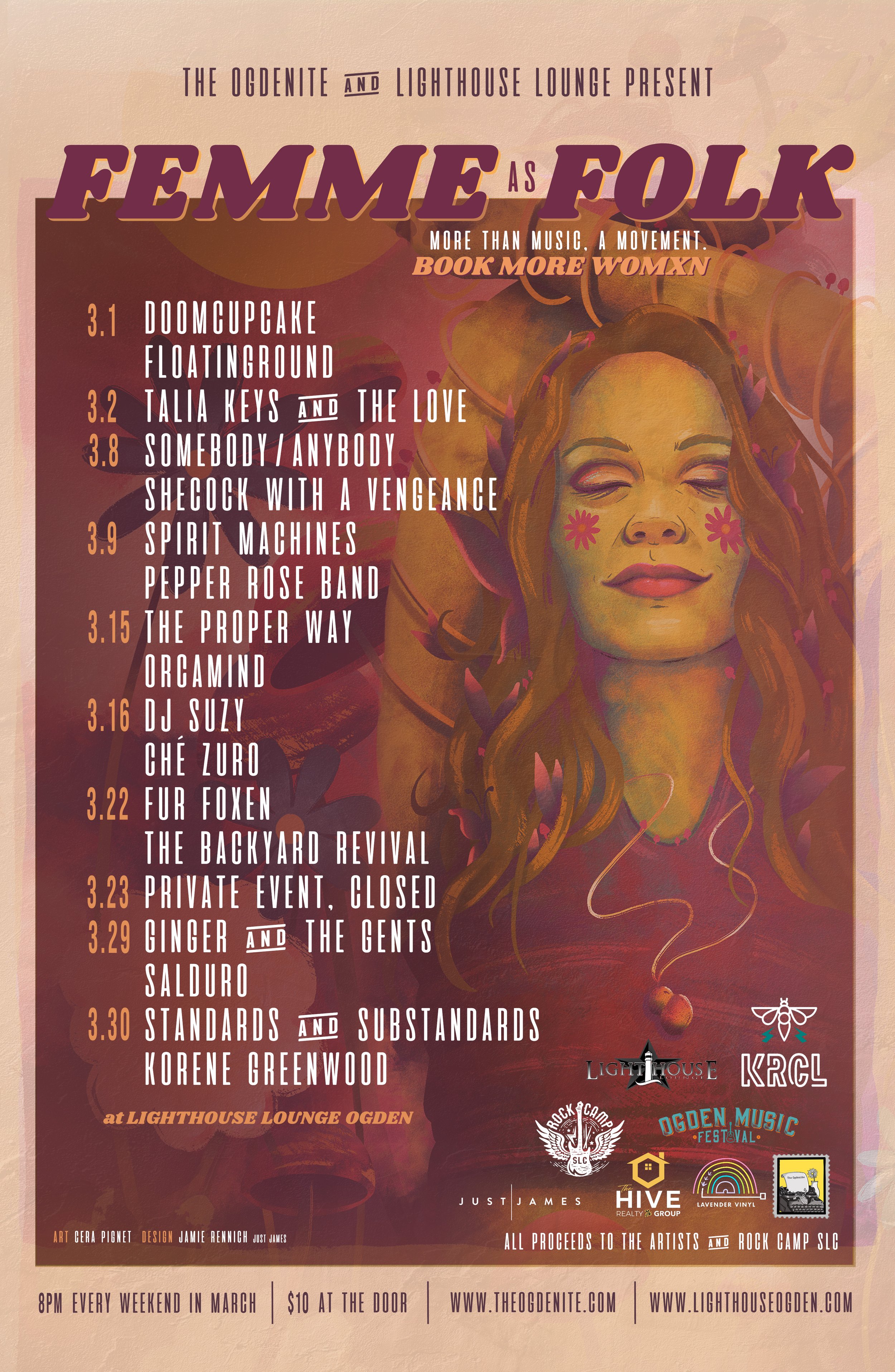This promotional flyer presents "The Ogdenite and Lighthouse Lounge Present: Femme as Folk – More Than Music, A Movement, Book More WOMXN," featuring a series of events. The background is a light beige or pink with purple lettering. A prominently featured image depicts a woman with long brownish-red hair, wearing a purple tank top, her hands raised leisurely over her head, and flowers drawn on her cheeks. 

The left side lists the performance dates throughout March: 3-1, 3-2, 3-8, 3-9, 3-15, 3-16, 3-22, 3-23, 3-29, and 3-30. Performers include Doom Cupcake, Floating Ground, Talia Keys and the Love, Somebody Anybody, Shecock with Vengeance, Spirit Machines, Pepper Rose Band, The Proper Way, DJ Susie Chisoro, Fox in the Backyard, Revival, Private Event Closed, Ginger and the Gents, Saldaro Standards and Substandards, and Kareem Greenwood.

The bottom of the flyer highlights, "8 p.m. every weekend in March, $10 at the door. All proceeds to the artists and Rock Camp SLC." A website for further details is also provided.